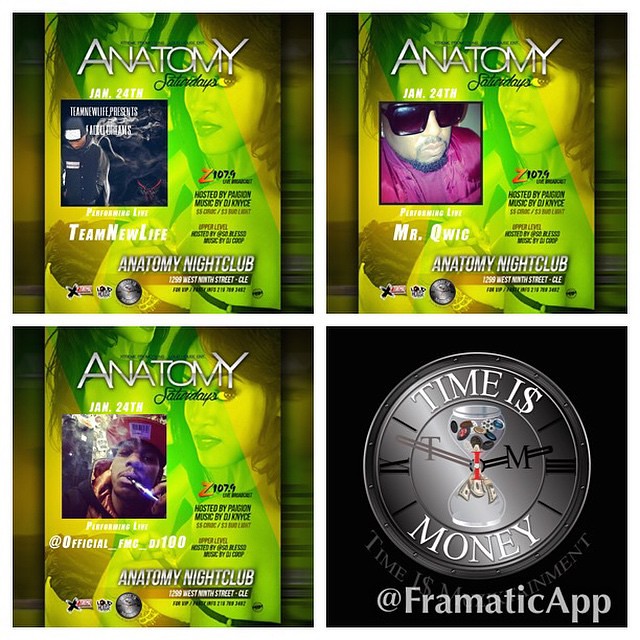The image is a square graphic divided into four equal parts by white lines forming a plus shape. Three of the quadrants feature green-themed advertisements promoting "Anatomy Saturdays" at the Anatomy nightclub in Cleveland. Each of these advertisements highlights different performers: one promoting "Team New Life," another featuring "Official FMC," and the third showcasing "Mr. Quick (Kwic)". All performers are depicted in these sections, showing pictures of African-American individuals against a green backdrop. Additionally, the event is hosted by Z107.9's Pagan with music by DJ Nice (Knyce). The fourth quadrant, located in the bottom right corner, deviates from the green theme; it has a black background and displays a silver watch alongside the phrase "Time is Money." This quadrant also mentions the "Frmatic App" and displays elements like money and tokens around a clock.